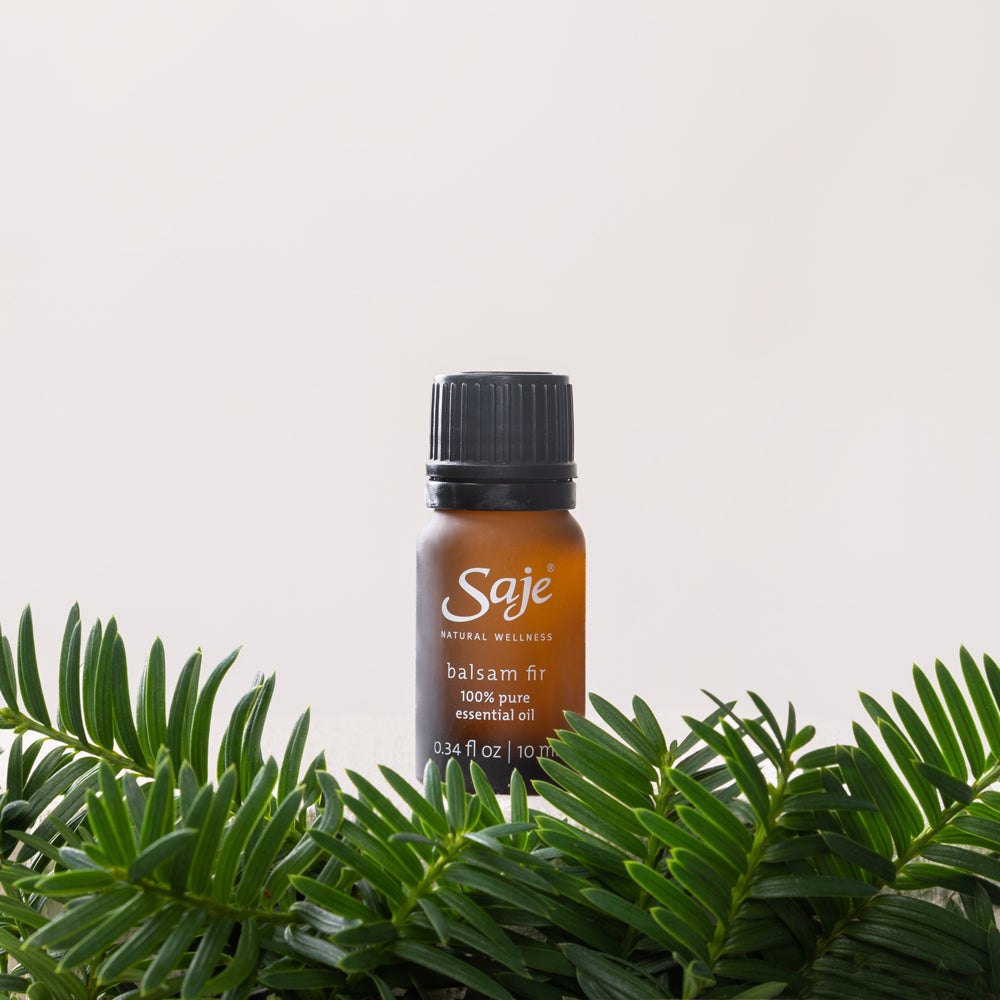This well-lit advertisement photo showcases a small, brown bottle of Saje Natural Wellness Balsam Fir 100% Pure Essential Oil, containing 0.34 fluid ounces (10 milliliters). The bottle, prominently positioned at the center of the image, features a black, ribbed cap and white lettering detailing the product's name and specifications. The color of the bottle resembles tree sap or honey. Surrounding the bottle in the foreground are numerous evergreen branches, adding a natural element that frames the product. The background is a clean white, making the details on the bottle and the contrast of the evergreen foliage stand out vividly. There are no shadows cast by the bottle, emphasizing the clear and pristine presentation of the essential oil.